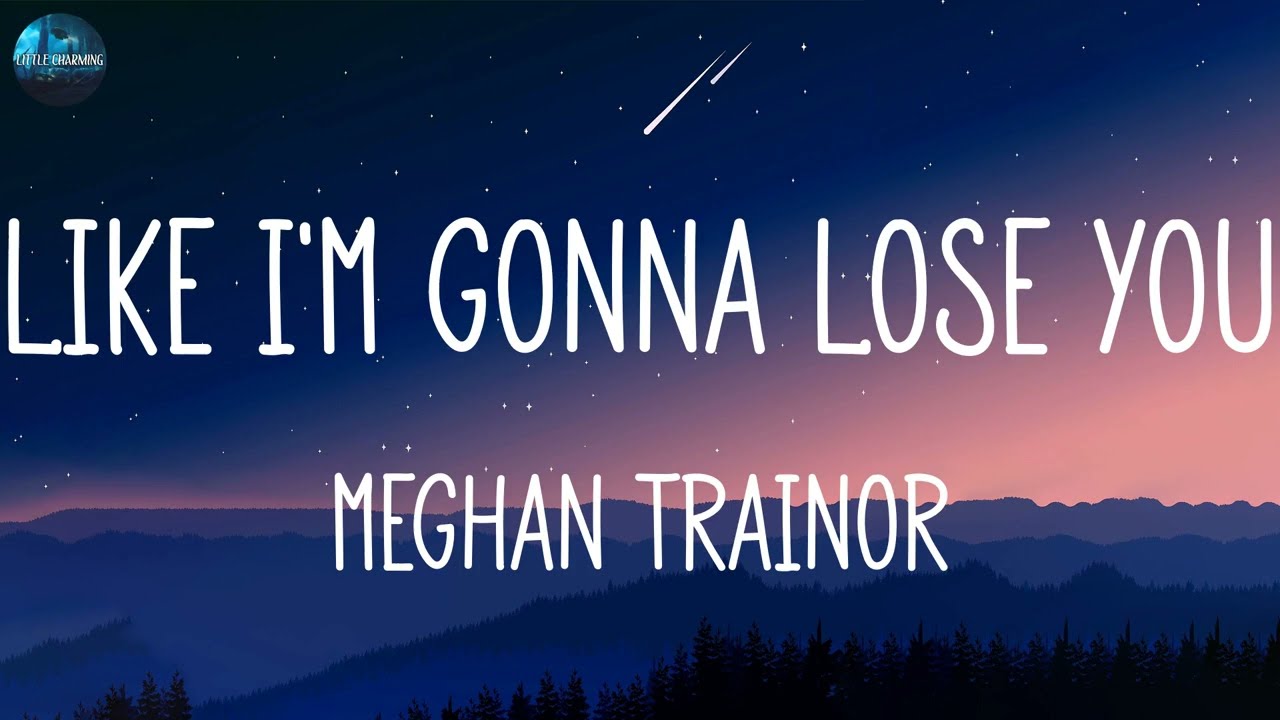This is an animated cover image for the music video of "Like I'm Gonna Lose You" by Meghan Trainor. The background features a nighttime scene of the Great Smoky Mountains, depicted in various shades of blue. Silhouettes of trees span across the bottom, while the sky transitions from a pinkish-orange near the horizon to a deep blue at the top, dotted with stars and a couple of shooting stars. White uppercase text boldly states the song title, "LIKE I'M GONNA LOSE YOU," with Meghan Trainor's name displayed in slightly smaller letters beneath it. There is also a small, unreadable, charming logo in the upper left corner of the image.